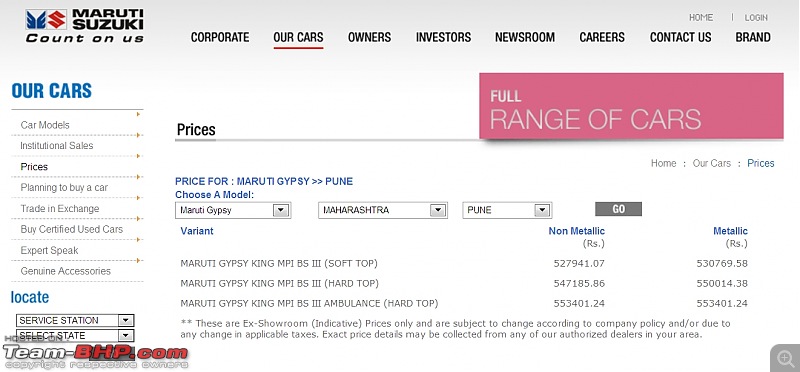The webpage dedicated to Maruti Suzuki is structured with the brand name 'Maruti Suzuki' prominently displayed on the left in black text, accompanied by the tagline 'Count on us' below it. Adjacent to the name, there is a small blue feather-like icon with a red 'S'. The navigation menu features categories such as Corporate, Our Cars, Owners, Investors, Newsroom, Careers, Contact Us, and Brand, all in black text with 'Our Cars' highlighted in red.

In the upper right corner, there are options to 'Home' or 'Log In' in gray. On the left sidebar, 'Our Cars' is prominently displayed in blue, followed by a list that includes Car Models, Institutional Sales, Prices, Planning to Buy a Car, Trade-In, Exchange, Buy Certified Used Cars, Expert Speak, and Genuine Accessories, all in gray text with a small gold arrow pointing to the right.

At the bottom of the sidebar, 'Locate' is displayed in blue. Below this section, banners are visible, including one labeled 'Service Station' followed by 'Select State,' with another partially visible banner reading 'Team BHP com,' where 'BHP com' is in red and 'team' in white. To the right, there's a section titled 'Prices' with a fine gray line separating it.

In the center of the page, a large pink banner reads 'Full Range of Cars' in white text, followed by detailed pricing for Maruti Gypsy in Pune. The options to 'Choose a Model' are in blue with dropdown menus for 'Maruti Gypsy,' 'Maharashtra,' and 'PUNE,' each accompanied by a downward arrow.

Below these dropdowns is a black banner containing the word 'Go.' Above that, there are navigation options for 'Home,' 'Our Cars,' and 'Prices,' with 'Prices' highlighted in blue. The page lists three variants of Maruti Gypsy King cars: Soft Top, Hard Top, and Ambulance Hard Top, further categorized into 'Non-Variant' and 'Non-Metallic,' followed by a series of numeric listings.

At the bottom, a disclaimer with two asterisks states: "These are ex-showroom indicative prices only and are subject to change according to company policy and/or due to any changes in applicable taxes. Exact price details may be collected from any of our authorized dealers in your area."